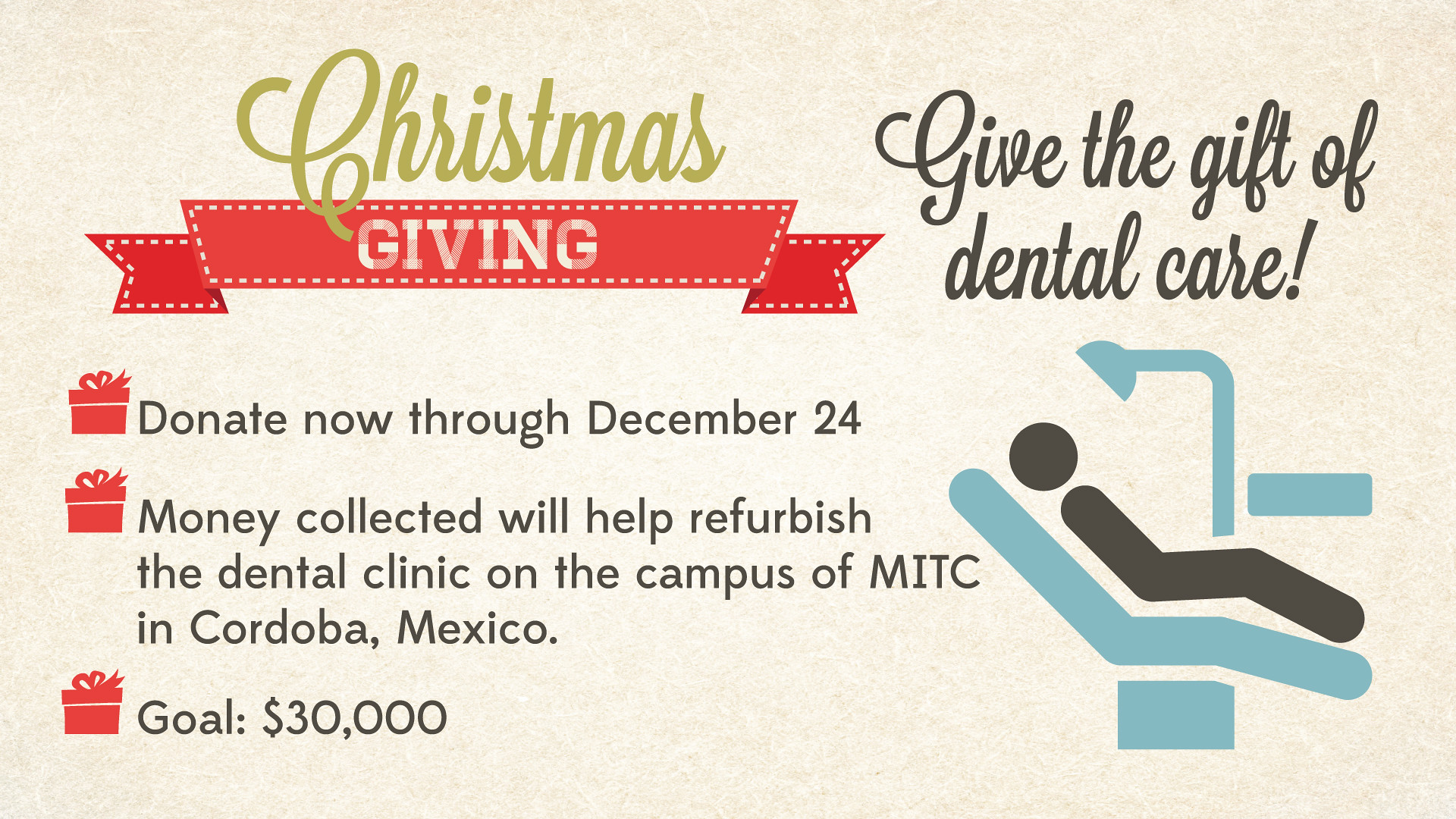Displayed on a beige postcard, this advertisement encourages holiday donations for a dental care cause. At the top left, the words "Christmas Giving" are prominently featured, with "Christmas" in elegant cursive gold letters and "giving" in bold text on a festive red wavy ribbon. The top right message, "Give the Gift of Dental Care," is written in black text. Below it, a clip art illustration depicts a person reclining in a dental chair, complete with an overhead light and a side tray. 

To the left of the illustration are three bullet points, each marked with a red gift icon. The bullet points read:
1. "Donate Now through December 24th."
2. "Money collected will help refurbish the dental clinic on the campus of MITC in Cordoba, Mexico."
3. "Goal: $30,000."

The card seems to be intended for distribution at dental offices to solicit funds for the refurbishment of the dental clinic, providing donors with a clear and festive message of how they can contribute to the cause.